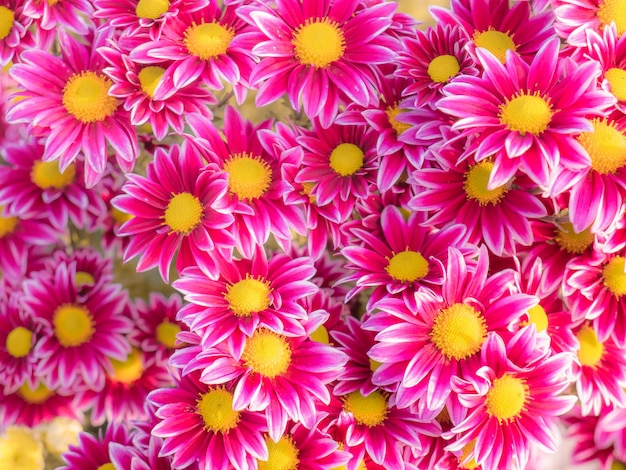This detailed photographic image captures a top-down view of approximately 30 chrysanthemums, all exhibiting vivid pink petals with white borders that frame a bright yellow center, from which protrude tiny, yellow spikes. The flowers are uniformly sized and predominantly occupy the frame, with their roughly ten petals each creating a visually rich and textured composition. These blooms, seemingly scattered in a natural and somewhat random arrangement, are set against a subtle backdrop of green foliage, further enhancing the vibrant pink and yellow hues. While it remains ambiguous whether the photograph was taken indoors or outdoors, or if it's a digitally rendered artwork, the image compellingly captures the dense, colorful array of chrysanthemums in what appears to be a flourishing flower bed. No text is present within this intricate display of floral beauty.